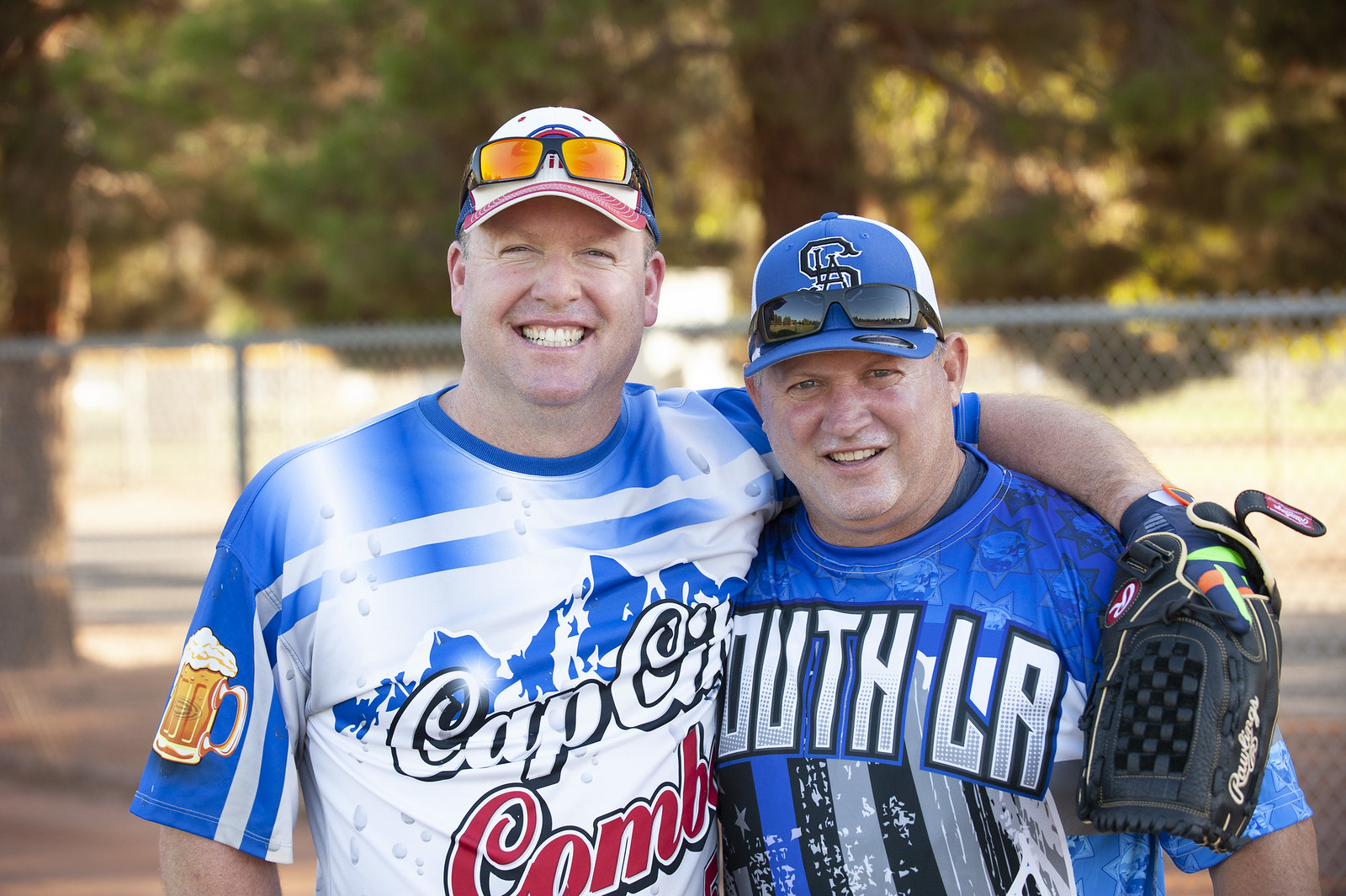This is a detailed photograph taken on a sunny day of two baseball players standing side by side, smiling at the camera. The man on the left, a white male, has his arm around the man on the right and is holding a large black leather catcher's mitt. He is wearing a white baseball cap with orange mirrored sunglasses resting on top and a blue and white jersey that features a beer mug on his left sleeve and mountains on the chest. The visible text on his jersey appears to say "Cap City COMB," though part of it is cut off. The man on the right, also a white male, is slightly smaller and is wearing a blue baseball cap with black sunglasses resting on the bill. He is dressed in a blue jersey with partially visible text "OUTH" and "LA." Opaque green leaves from tall trees, backlit by sunlight streaming through the branches, can be seen behind a tall metal chain-link fence in the background, giving the image a cheerful, sunlit ambiance.